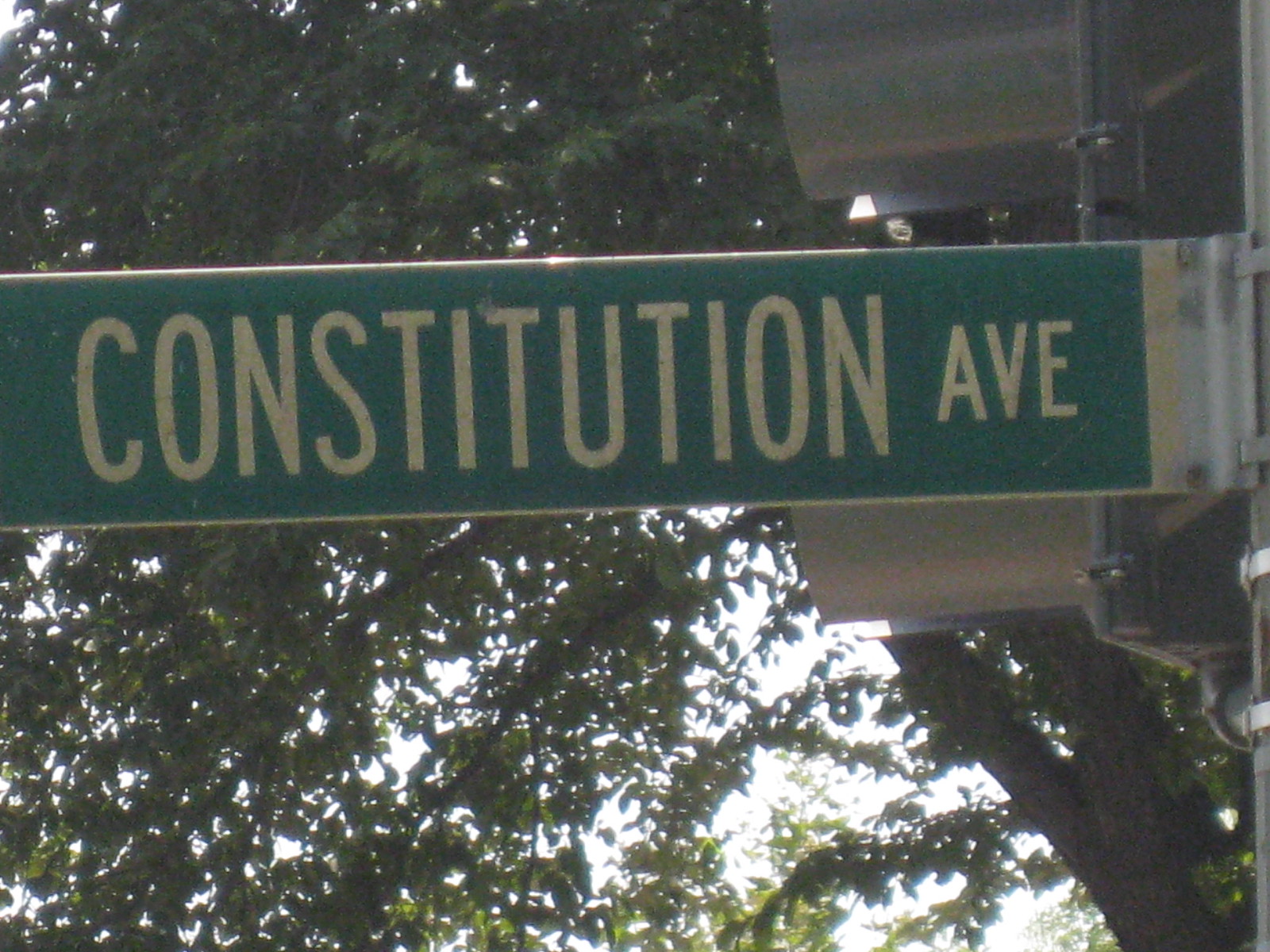This is an upward-angled photograph showcasing a green street sign with white lettering that reads "CONSTITUTION AVE." The sign is affixed to a sturdy metal pole. Below the sign, two traffic lights are visible, partly obscured by large metal housings. A prominent walk/don't walk signal is also discernible beneath the sign, although its light status is unclear. Dominating the background is a massive, leafy tree through which patches of bright, clear sky peek through. The scene suggests a sunny day, capturing the vibrant green foliage and the clean, cloudless sky. The image composition focuses on the urban elements against the backdrop of nature, providing a vivid street-level perspective.